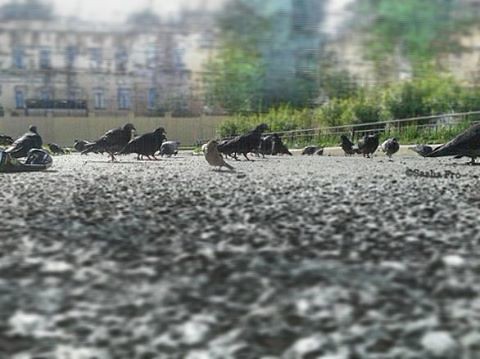This highly detailed colour photograph captures a low-angle, almost ground-level view of a stony or asphalt surface, possibly a street or car park. The focal point is a group of approximately a dozen birds, predominantly pigeons with assorted other species, situated in a loose line slightly above the midline of the frame. These birds, varying from dark gray to lighter brown hues, appear to be either feeding or casually standing around.

The background, rendered with a bokeh effect, blurs out its elements, but you can discern various structures and foliage. To the right are trees and bushes, possibly fenced off. On the left, a large, multi-windowed building, likely an apartment complex or low-rise city structures, looms in the distance. The sky above gives an impression of overcast conditions with patches of blue barely visible.

The photographer, whose name appears to be Sasha Froh, has successfully utilized this perspective to draw attention to the birds and the detailed texture of the pavement while subtly incorporating the park-like cityscape in the background. The setting hints at an urban environment bordering on natural elements, with hints of an old-world charm reminiscent of European cities like Venice or Italy.